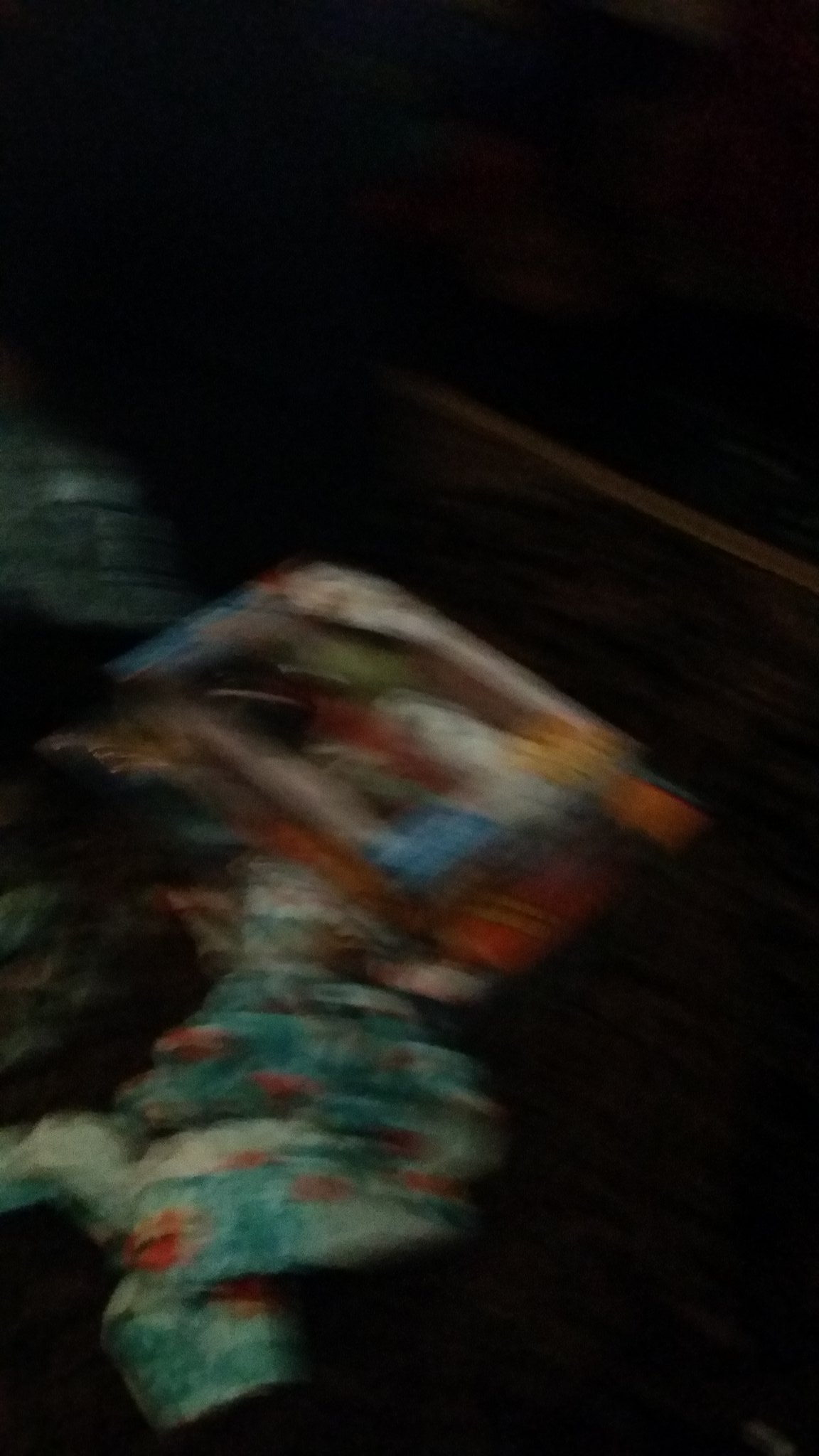The image features a very dark black background with an overall blurry and indistinct depiction, which gives it a painted and hazy appearance. At the top of the image, a square about three to four inches long stands out, filled with areas of white, yellow, and red, suggesting a 3D effect with an additional layer of red behind it. Below that, there is a thin, long rectangular piece in green and white, connecting to what appears to be a bundle shaped like a wrapped blanket with green, red, and a hint of white. This bundle tapers into a cylinder shape culminating in a very short rectangle. Other visible elements in the blurred composition include pink, blue, orange, black, and brown hues blending together, resembling a pile of clothes or a combination of various cloth-like objects.